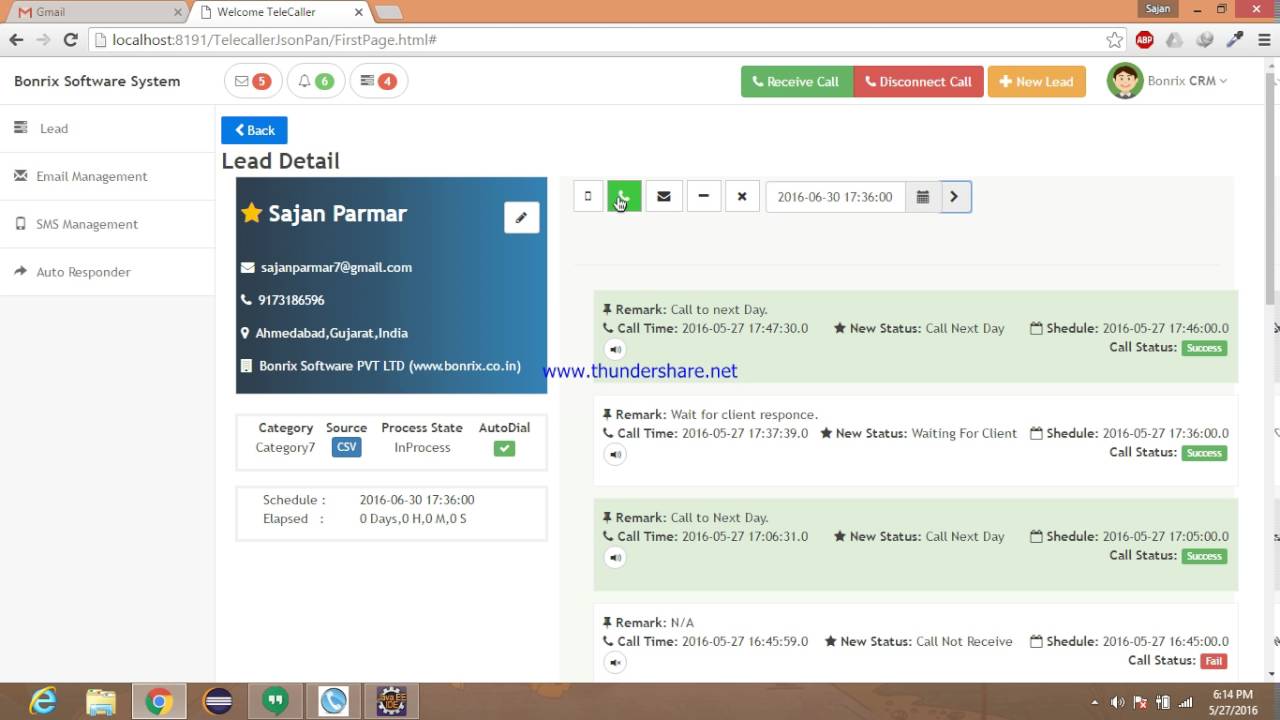The image is a detailed screenshot of a computer screen, presented in a left-to-right horizontal layout. The background incorporates the white hue typically associated with computer interfaces. At the top of the screen, there are several open tabs, including a Gmail tab and a "Welcome Telecaller" tab. Below these tabs, there is an orange horizontal line, indicating the active window’s frame. 

On the upper right corner of the window, the icons for minimize, maximize, and close are visible. Moving to the left, the navigation bar features back and forward arrows, a refresh button, a search bar, and additional icons on the right side.

Directly beneath the search bar, the Bonrex software system interface is displayed. This includes sections for emails, alertifications, and notifications, each with a numeric indicator showing the number of items. Further down, the Bonrex logo and labels are seen for "Lead Email Management," "SMS Management," and "Auto Responder."

Towards the top right of the screen, there are buttons for "Receive Call," "Disconnect Call," and "New Lead Options." Adjacent to these buttons, there is a profile picture associated with Bonrex CRM. A blue "Go Back" button is also present. The lead details for an individual named Sajan Parmar are shown, including remarks, call times, interactions with the client, and follow-up actions like "Call next day."

At the bottom of the screenshot, the typical elements of a computer’s taskbar can be seen, featuring icons for Internet Explorer and Chrome, as well as the time and date on the right-hand side.